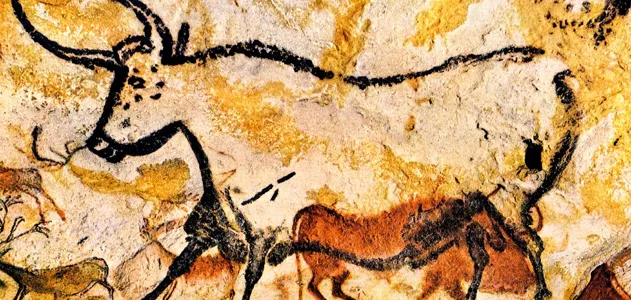This image depicts a cave painting on a rough, blotchy rock surface with various shades of gold, brown, and tan. Dominating the scene is a large black charcoal-like outline of an ox facing left, its intricate details showing large horns, eyes, nose, and legs, with some additional black markings accentuating its features, especially prominent on the lower part. Beneath the ox, painted in brown pigment and oriented in the opposite direction, is a smaller animal resembling a boar with darkened areas around its eyes and legs. In the bottom left corner of the painting, partially off the edge, are smaller, deer-like animals characterized by their unique body types and distinct antlers, adding to the intricate detail of this ancient artwork.